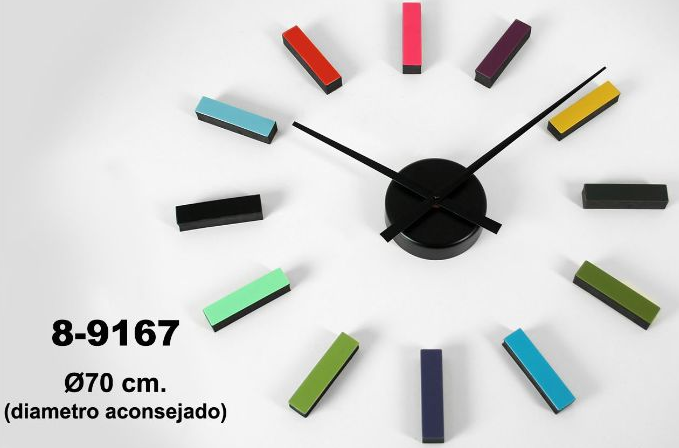The image depicts a modern clock mounted on a white wall, viewed from a slight upward angle. In the lower left-hand corner of the photo, the text "A-9167," followed by a symbol of a zero with a slash through it, "70cm," and the words "(DIAMETRO ACONSEJADO)" appear in black. The clock itself is unconventional, featuring no numbers, but instead, an array of small, rectangular bars to denote the hours. These bars are color-coded as follows: the bar at 12 o'clock is red, followed by brown, yellow, black, dark army green, blue, black, green, light green, black, turquoise, and finally, red again at 11 o'clock. The center of the clock is marked by a black, 3D-like circular disk, from which two slender, black hands extend to indicate the time. Based on the hands' positions, the hour hand points just past 10, while the minute hand is near 9, suggesting the time is approximately 10:09.